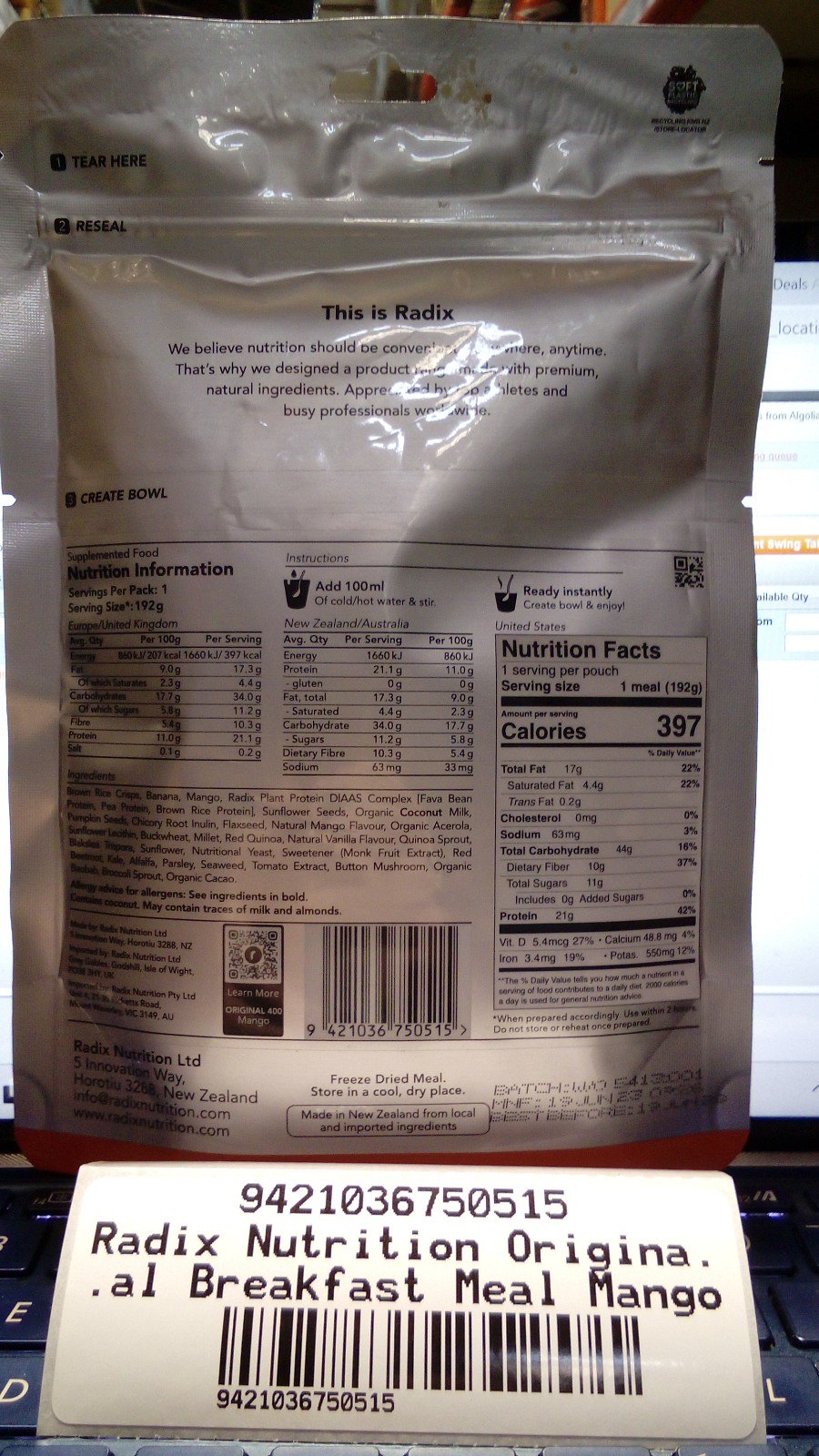This image depicts the back of an unopened silver bag, still securely sealed. At the top of the bag, the word "Radix" is prominently displayed. Below this title, there is a blurb that is not clearly legible. Underneath the blurb, detailed nutritional information is presented within a nutrition facts box, accompanied by several smaller, less discernible boxes. The ingredients list is also present but printed too tiny to read. Toward the bottom of the bag, a barcode and a QR code are visible. The bag indicates that the product is made in New Zealand, although the specific location is out of focus. Prominently displayed at the bottom is a large label that reads, "Radix Nutrition Oregona Breakfast Meal Mango."